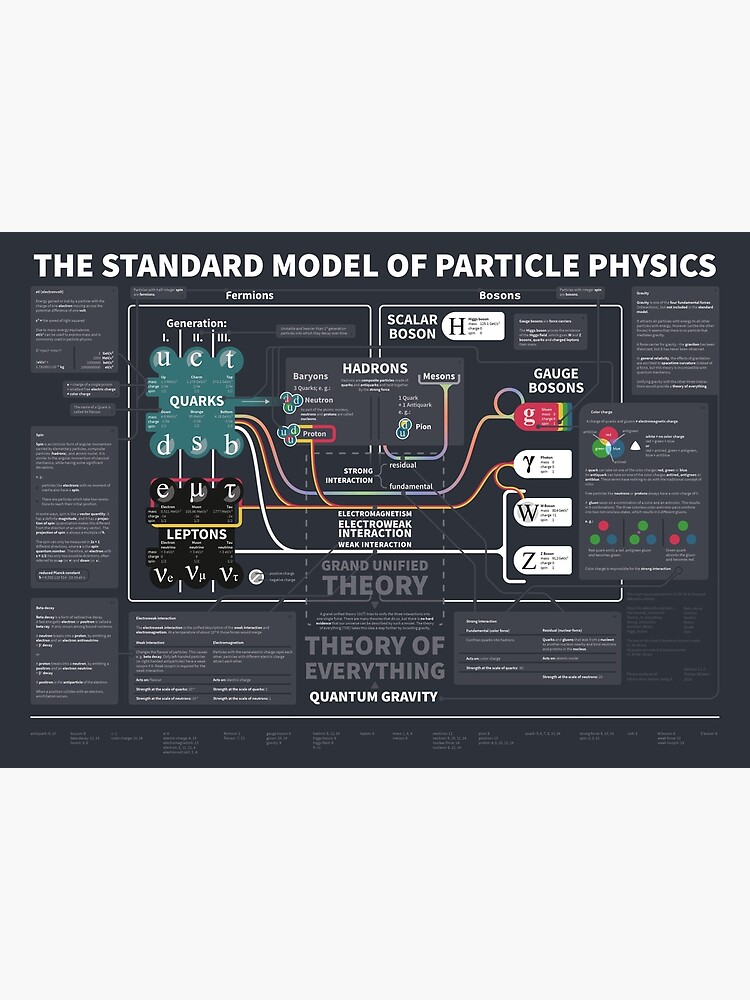The image is a computer-generated diagram titled "The Standard Model of Particle Physics." Although the image is of limited size, making most text difficult to read, the diagram is set against a black background with predominantly white text. The legible text includes terms such as "Grand Unified Theory," "Theory of Everything," and "Quantum Gravity." The diagram appears to illustrate the interconnections between various particles through intricate flowcharts, depicting a highly detailed and scientific representation of particle interactions and theoretical frameworks.